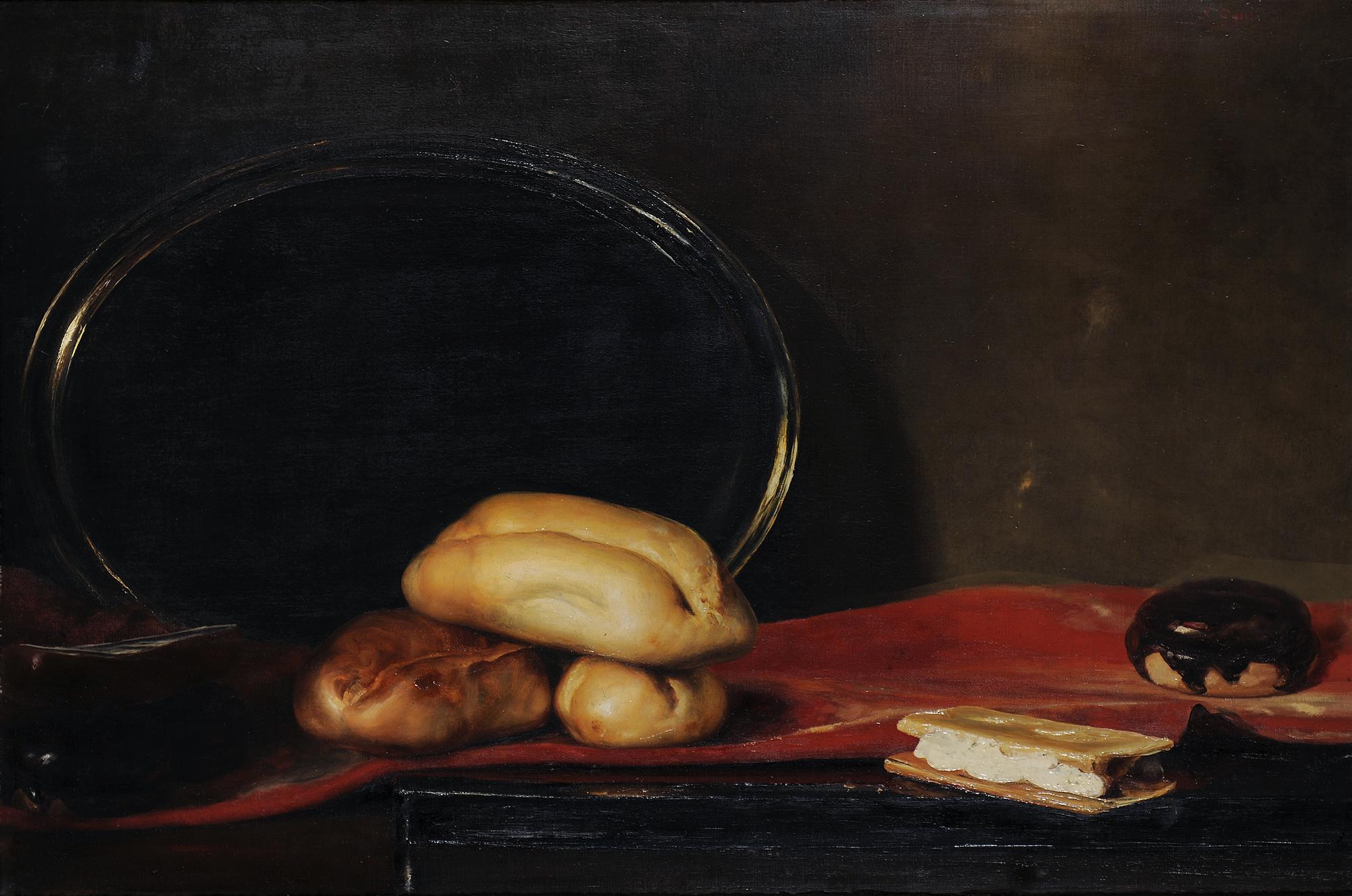The image portrays a highly realistic painting of an arrangement of breads and pastries on a red cloth atop a dark-colored table. Central to the composition are three breads: two smaller ones lying side by side, and a larger one set perpendicularly across them, giving the illusion of a figure in a fetal position at first glance. One of the smaller breads features a browned or sauced top layer, while the larger one resembles a plain French loaf. Adjacent to this is a silver plate or mirror tilting diagonally in the background. On the table, there is also a Boston cream donut with chocolate spilling over its edges, and nearby, a graham cracker s'more sandwich with white icing in the middle. The backdrop of the scene is characterized by a dark, brownish wall, adding depth to the overall somber yet rich visual.